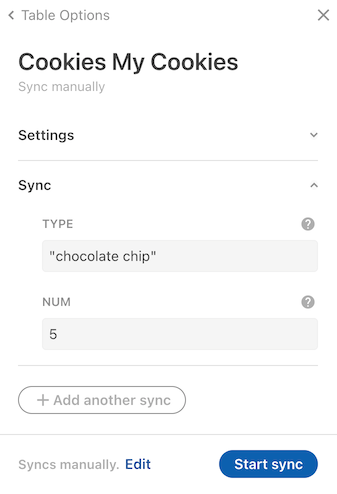The image depicts a website interface focused on table synchronization options. At the top, the caption "Table Options" is displayed in light gray, accompanied by an 'X' icon to the right for closing the options. Below, the title "Cookies" is prominently written in dark black, followed by the subtext "Sync Manually".

On the right, there's a "Settings" label with a downward arrow indicating a dropdown menu. Underneath, the word "Sync" appears with an upward arrow next to it. Further down, a section labeled "Type" features a question mark on the right side, next to a gray bar labeled "Chocolate Chip."

Below, another section labeled "NUM" also has a question mark on the right, beneath which is a gray box containing the number "5". A light gray box segments this section from the rest of the interface.

There is a large white box outlined in gray with the text "Add Another Sync" alongside a plus sign (+). The section continues with the options "Syncs Manually" and "Edit" highlighted in purple.

At the bottom, a prominent blue box with rounded edges is labeled "Start Sync," indicating the button to initiate the synchronization process.